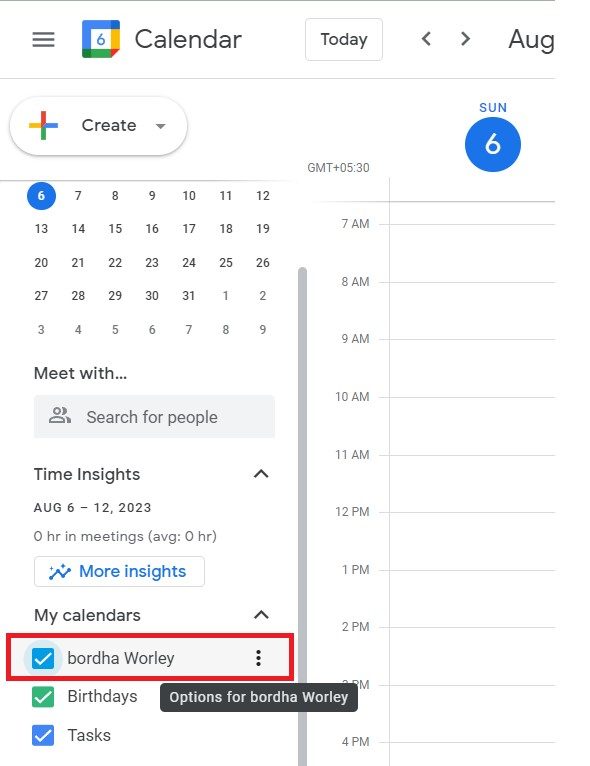The image is a smartphone screenshot of a Google Calendar web page. At the top of the interface, there is a hamburger menu icon, followed by the Google Calendar logo and the word "Calendar." To its right, there is a "Today" button, flanked by left and right navigation arrows. The month "August" is prominently displayed, indicating the current view. 

Below this header, there is a "Create" button with a dropdown arrow, allowing users to create new calendar events. The date "6th" is highlighted, suggesting it is the selected date, and this confirms it is the month of August, as mentioned above.

The screen is split in half with the right section showing timestamps in GMT +5:30. Below the calendar controls, there is a "Meet with..." search field where users can find people to schedule meetings with. Hovering near this section is a dropdown box for "Time Insights," showing data from August 6th to 12th, 2023. The insights indicate "0 hours in meetings" and an average of "0 hours," with an option for "more insight highlights."

Further down, there are tabs for "My Calendars," which is a dropdown showing selected calendars including "Birthdays" and "Tasks." To the right of these tabs, timestamps for Sunday, the 6th are displayed in vertical order from 7 AM through 4 PM, marking the hours when events can be scheduled.

This detailed visual layout captures the essential functionalities and user interface elements of the Google Calendar on a smartphone screen.